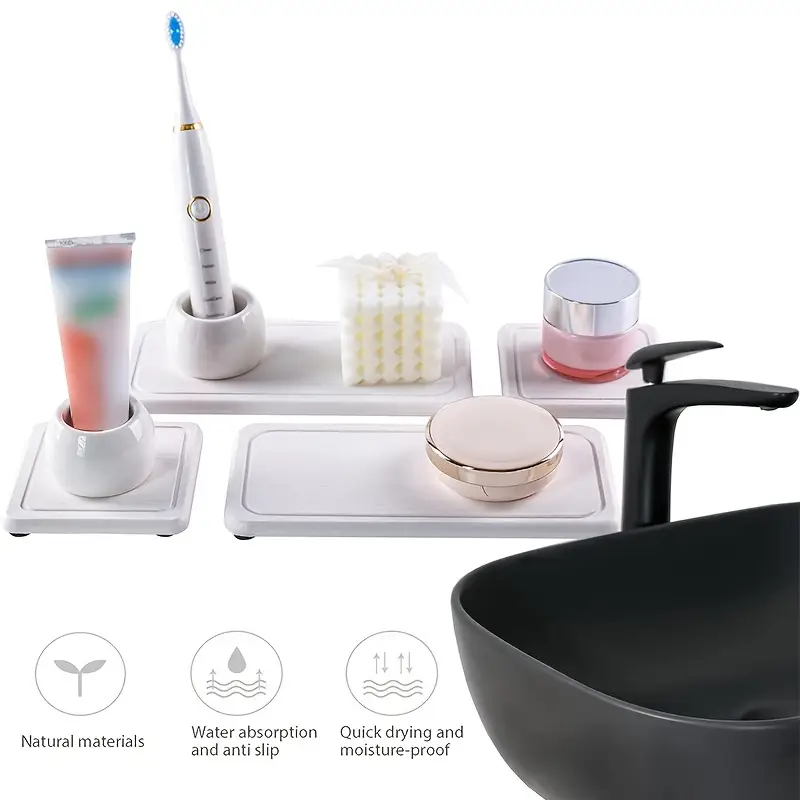This image features an advertisement set against a pristine white background, showcasing organizational pads for a bathroom countertop. In the bottom right corner, there is a sleek black sink with a matching black faucet. Scattered across the scene, positioned on white rectangular and square pads, are various bathroom essentials. These include an electric toothbrush in a white holder, a tube of toothpaste, several bottles of lotion and makeup dispensers, and a distinctive circular container with a pink item inside. Notably, each item is arranged meticulously on its individual pad that emphasizes the product's organizing function. Displayed text below the pads highlights the features: "natural materials," "water absorption," "anti-slip," "quick-drying," and "moisture-proof," reinforcing the practical benefits of these organizational elements for a tidy bathroom setup.